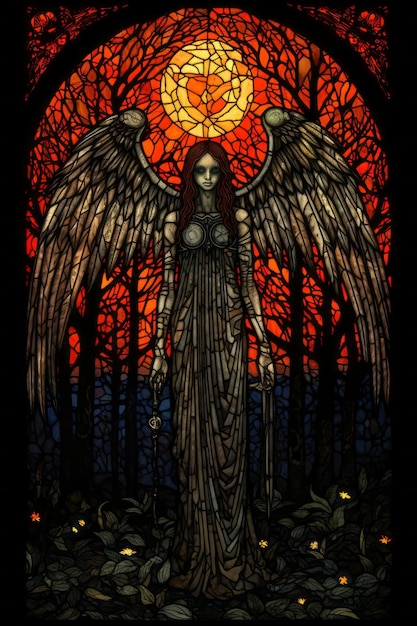The image appears to be a detailed illustration with a gothic, slightly horror aesthetic, resembling a stained glass window. It depicts a female dark angel with auburn hair and a very pale, almost lifeless complexion. Her dark eyes are downcast, giving her a somber appearance. She dons a long, lacy dress with scattered sleeves and wields objects in both hands, which are difficult to identify but may be swords. Behind her, large wings spread out, structured to be longer on the sides and shorter in the middle.

She stands amidst a forest, surrounded by trees with intertwining branches devoid of leaves, creating a stark, moody ambiance. The ground at her feet is scattered with small light-colored leaves or flowers. The background features a vivid blue near her legs, leading up to a reddish-orange sky. Above her, an arch of stained glass showcases shades of yellow and orange, possibly representing the sun, further contributing to the intricate and elaborate stained glass motif.